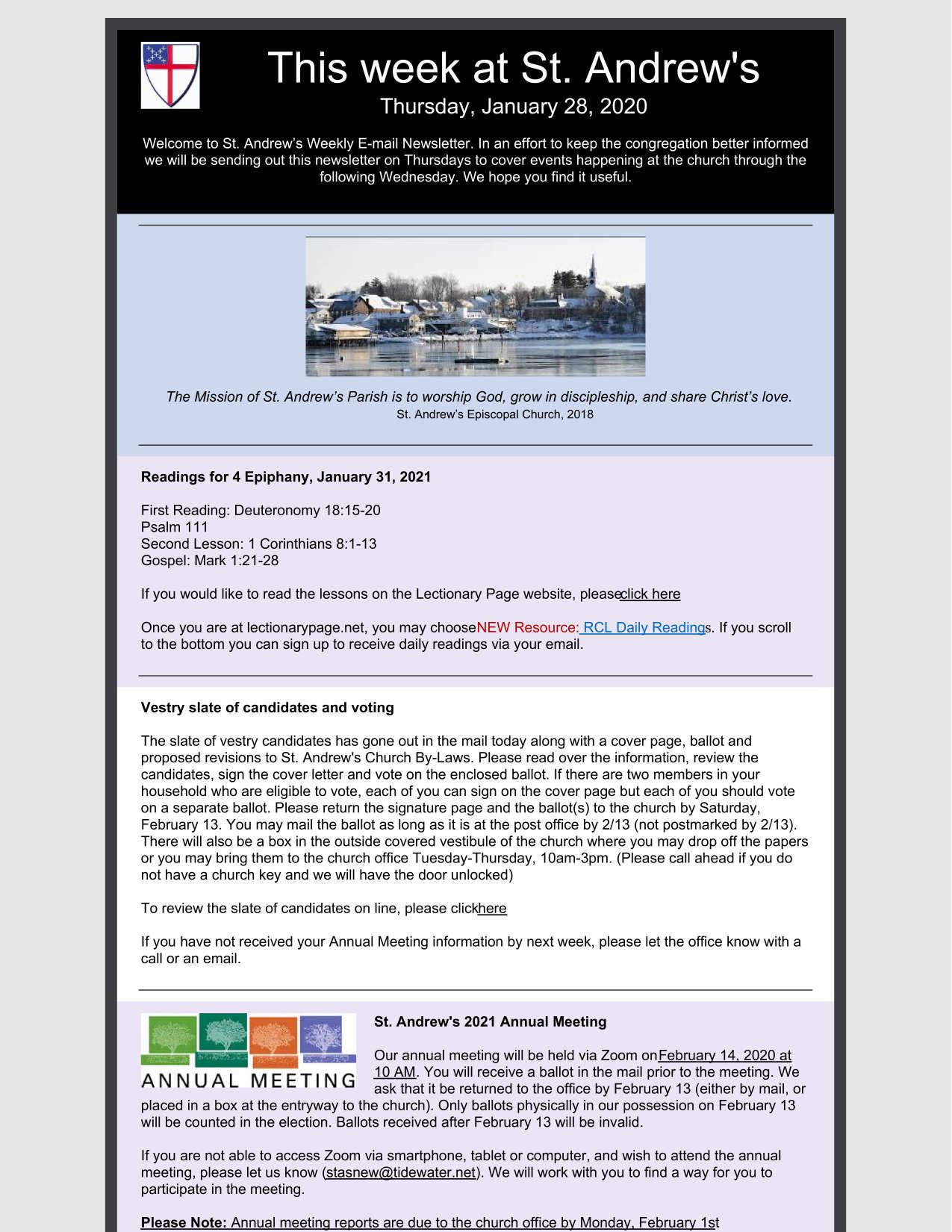**Caption:**

*This Week at St. Andrews - Thursday, January 28th, 2020*

At the top of the image is the text "This Week at St. Andrews" in white, below which is the date "Thursday, January 28th, 2020." On the left side, within a square, there is a shield featuring a red cross. The upper left quadrant of the cross is blue.

Beneath this, there is a photograph possibly depicting a large parking lot or outdoor area. Below the photograph, a caption reads: "The mission of St. Andrews Parish: to worship God, grow in discipline, and share Christ's love."

In the next section, there is a heading that reads "Readings for January 31st, 2021," followed by the text "new resource" in red. Below that, in blue and underlined text, it says "RCL Daily Readings."

The subsequent area is framed in a white box with the headline "State of Candidates and Voting," accompanied by an informational paragraph.

The final section is a light purple box with the text "St. Andrews 2021 Annual Meeting." The phrase "Annual Meeting" is prominently displayed in capital letters on the left side. Above this, there are four colored squares, each containing an image of a white tree. The squares are colored light green, dark green, orange, and purple respectively.